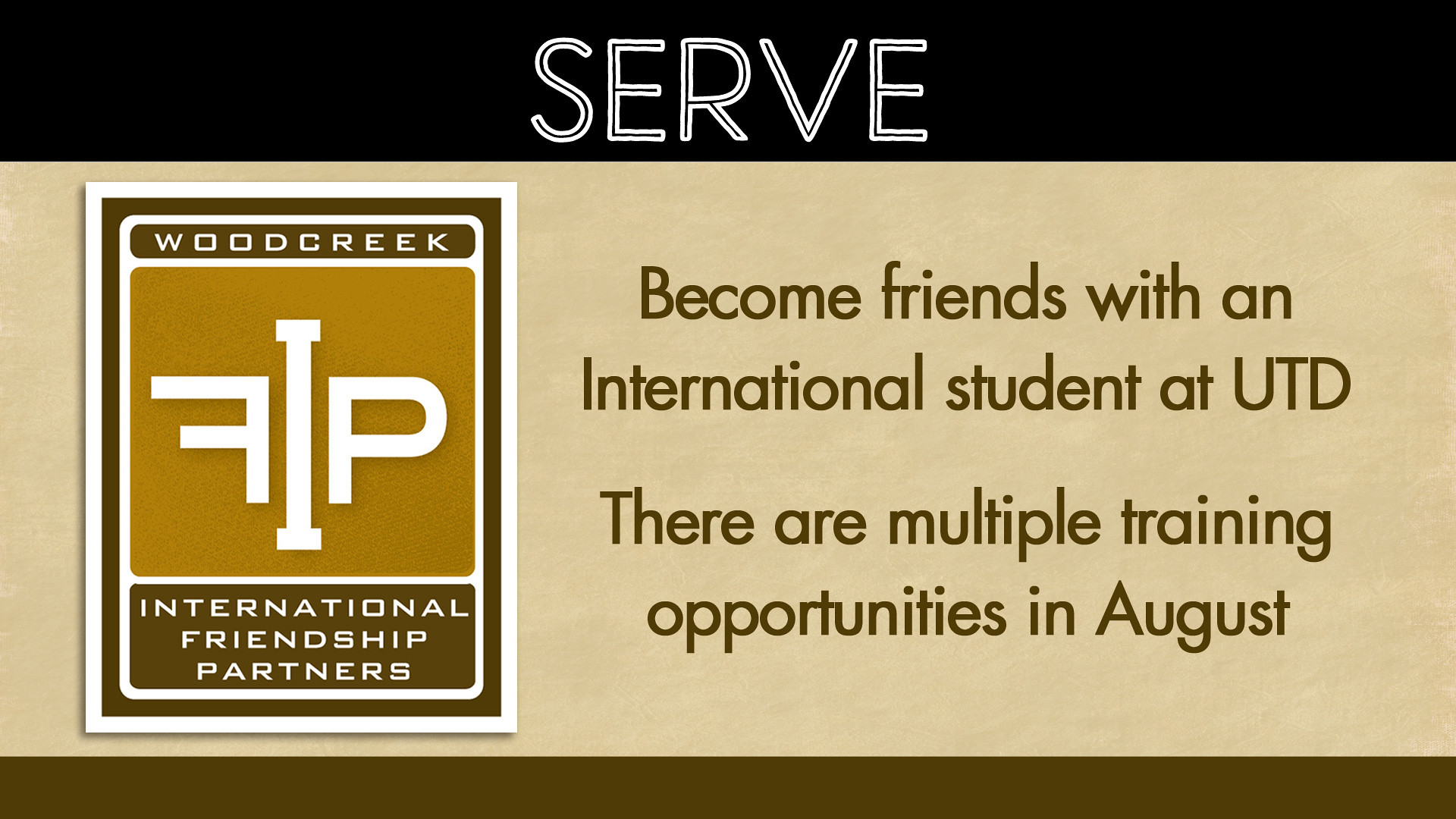The image depicts a predominantly beige business card with a prominent black band at the top. In white letters on this black band, the word "SERVE" is displayed. Below this, the central section contains a logo made up of varying tones of brown and white. The logo features the text "Wood Creek International Friendship Partners" with a backwards capital 'F', an elongated 'I', and a correctly oriented 'P' in white lettering amidst the browns. To the right of the logo, in dark brown text, the card reads: "BECOME FRIENDS WITH AN INTERNATIONAL STUDENT AT UTD," followed by, "THERE ARE MULTIPLE TRAINING OPPORTUNITIES IN AUGUST." At the bottom of the card, there is a thin dark brown border without any text. The overall design is clean and professional, geared towards promoting international friendship and engagement.